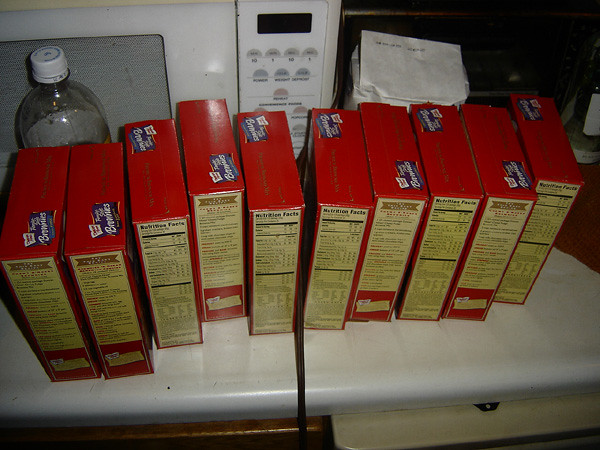In this image, we are peering into what appears to be a kitchen setting. The background reveals a microwave nestled against the wall and a clear plastic bottle filled with an unspecified liquid. The primary focus, however, is on an array of brownie mix boxes. Although the brand name isn't visible, each box prominently displays the word "brownie" on a blue label. There are precisely ten boxes of brownie mix lined up in a row. The nutritional labels on the boxes face the camera, but the text is too small to be legible from our viewpoint. These boxes rest on a pristine white countertop, giving the scene a neat and organized appearance.